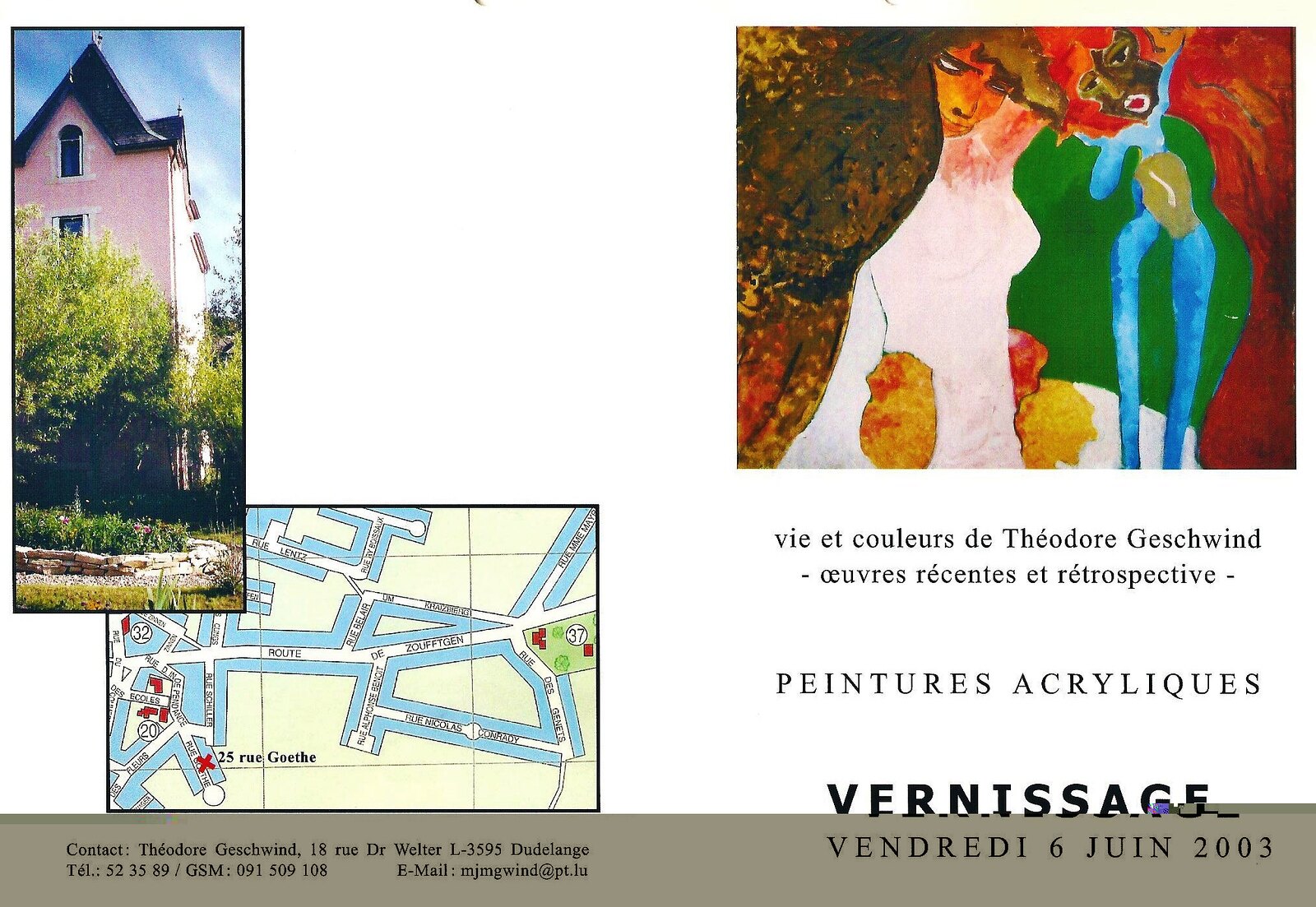This poster is an advertisement for a museum or gallery show featuring a variety of elements meticulously detailed to provide comprehensive information about the event. The poster is divided into three panels. The left panel showcases a vertical photograph of a picturesque pink house with a gray gabled roof, surrounded by trees, a bush, and a fence, suggesting the location of the event. 

Below this photograph sits a detailed map with a blue and yellow color scheme, marked with multiple street names including Rue Goethe, Rue de Zufken, Rue d'Aubelaire, and Rue de Genets, among others. Notably, the address “24 Rue Goethe” is clearly labeled, indicating a significant location related to the event.

In the top right corner of the poster, there is an abstract painting featuring two figures: a woman with an orange face, brown hair, and a naked body standing next to another figure with red hair, a blue body, and black skin. The accompanying text reads: "Vie et couleur de Théodore Geschwind, Oeuvres récentes et rétrospective, Peinture acrylique, Vernissage, Vendredi 6 juin 2003," translating to "Life and color of Théodore Geschwind, Recent and retrospective works, Acrylic paintings, Opening, Friday, June 6, 2003."

The bottom part of the poster includes essential information such as a border with details like telephone numbers, an address, an email address, ensuring prospective visitors have everything they need to attend the event.